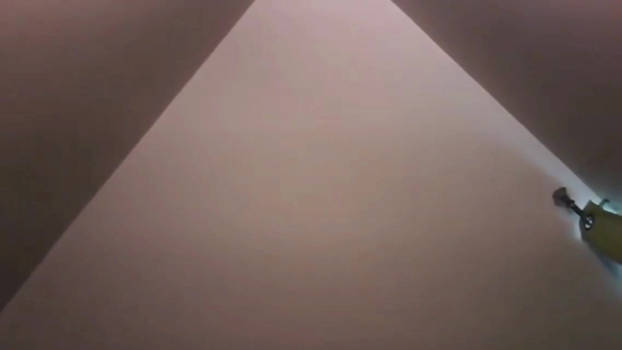This photograph depicts an intricate and somewhat perplexing scene. The landscape-oriented image features a fascinating interplay of colors and geometric shapes. A series of triangles create a mosaic-like pattern across the frame, though the arrangement does not seem deliberate. 

In the top left corner, a large brown triangle descends diagonally towards the bottom left, and then angles back upwards along the left side. A similar brown triangle occupies the upper right corner. Below and between these, a light brown triangle contrasts by pointing in the opposite direction, creating an interesting visual dynamic.

These individual triangles collectively form a larger, imperfect triangle with apparent gaps between them. This intricate assembly of shapes is the focal point of the pattern in the image.

Adding to the complexity, the right-hand corner of the photograph features an odd tool. This tool has a long, narrow handle with a small brush attached, appearing like it is brushing or scraping a surface. The tool is greenish and made of a plastic-like material, with a distinctive hole in the center where the brush is clipped.

Moreover, the tool emits a bright, green light, which illuminates part of the scene but feels oddly out of place in the otherwise organic setup. The purpose and function of this tool remain ambiguous, adding an enigmatic element to the overall composition.